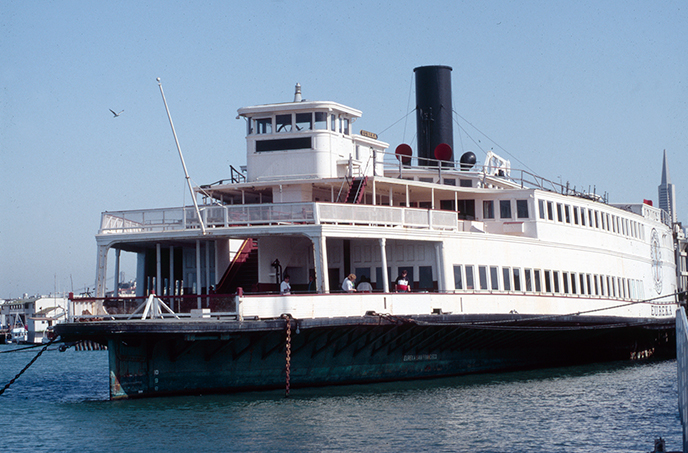This image showcases a large, two-story vessel, primarily white with numerous windows along its sides, indicative of a ferry or tourist boat. The vessel, docked on a clear, sunny day with minimal clouds, features a distinct black smokestack rising from its top. The upper level houses a control center or lookout cabin, elevated at the front, and offers a fenced-in deck area for passengers to enjoy views while sailing. The boat’s lower section is black, and several people are visible sitting and standing in the front deck area. In the background, you can spot a skyscraper, hinting at an urban setting, and additional sailboats. A bird is also seen flying in the upper left corner of the bright blue sky. The boat is moored with a visible rope extending from its front to the dock, completing the tranquil waterfront scene.